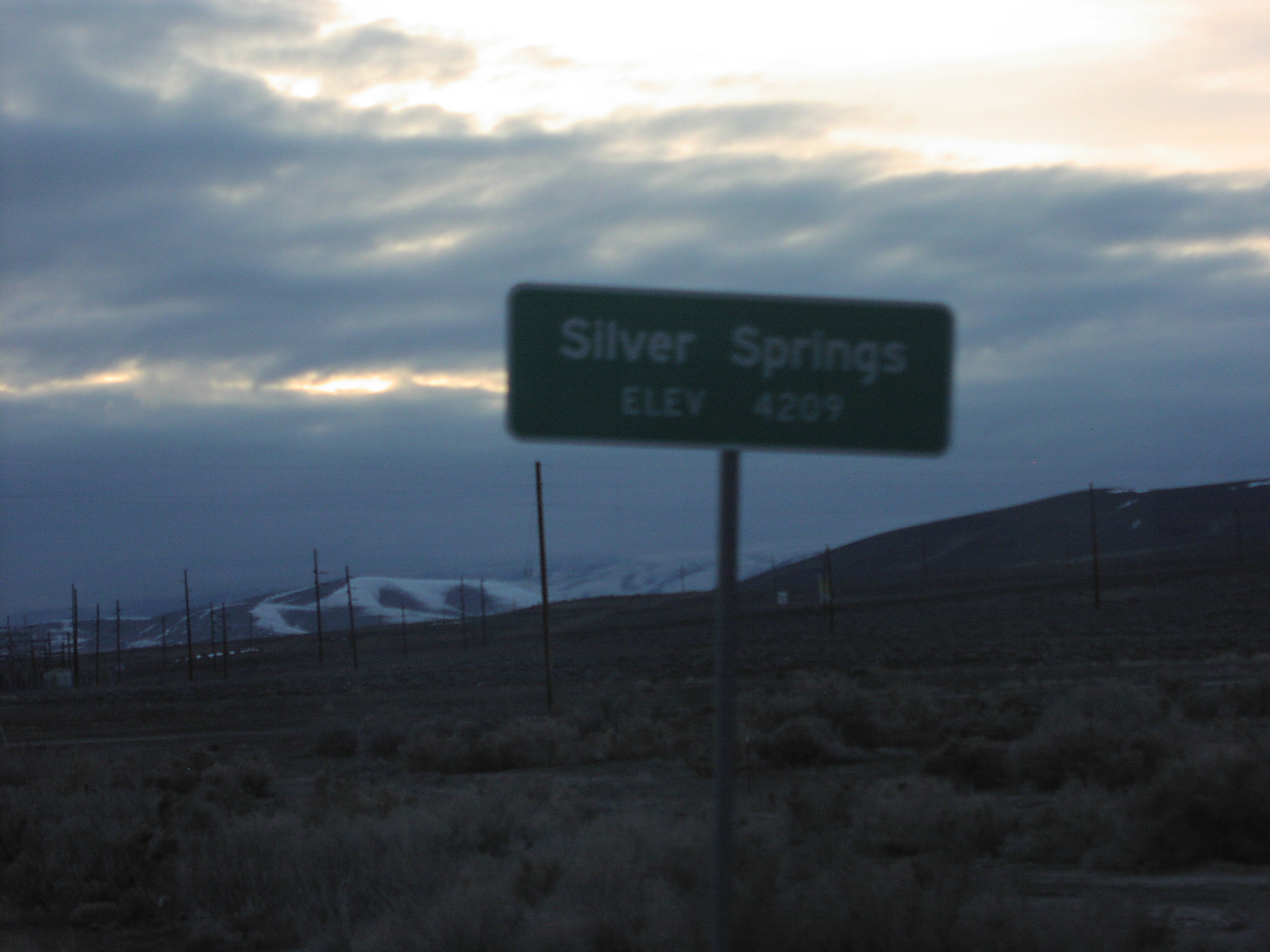This color photograph, likely taken from a moving car, captures a moody, dimly lit landscape either just before sunrise or around sunset. The image is slightly blurred due to the motion, with a weathered sign reading "Silver Springs, ELEV 4209" centrally positioned, slightly to the right. In the foreground, sparse desert brush hints at the arid conditions, while a snow-capped foothill rises to the right of the sign. Additional foothills stretch out in the background, creating a gentle, rolling horizon. Telephone poles punctuate the scene, adding to the desolate feel. The sky is dominated by a brooding dark gray, with beams of sunlight piercing through the clouds to the left of the sign and spreading across the upper portion of the image. The palette is muted, featuring soft browns, grays, and whites, contributing to the overall somber atmosphere.